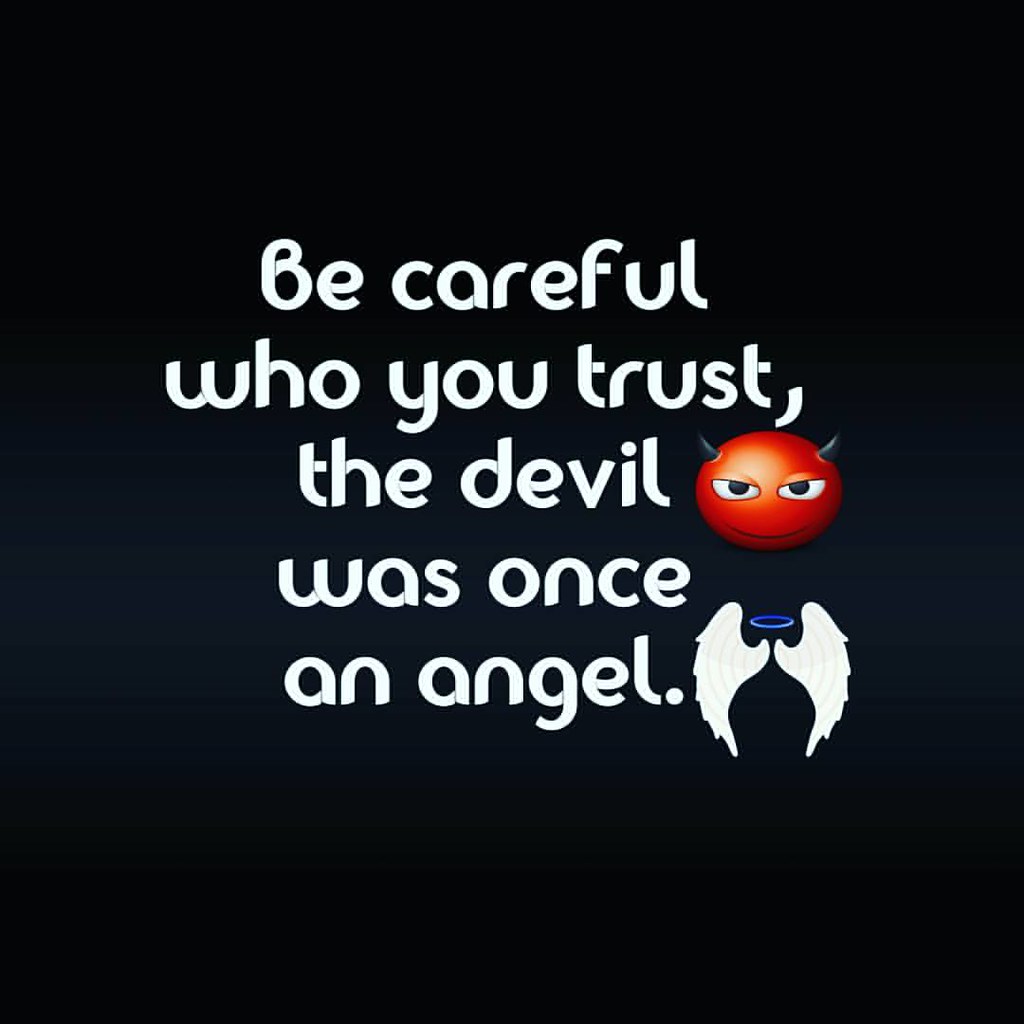The image features a predominantly black background that transitions to a dark gray in the middle, giving it an ombre effect. At the center, in bold white print, is the text: "Be careful who you trust, the devil was once an angel." The letters are all lowercase except for the "B" in "Be careful." Positioned to the right of the text, there's a cartoonish depiction of a red-faced devil head with black horns and black and white eyes. Directly beneath the devil image, there is a pair of white angel wings with a blue halo atop them. The overall composition is centralized and the text is presented in a casual, bubbly font, giving the image a meme or motivational graphic feel. The color palette includes black, dark gray, white, red, and blue.